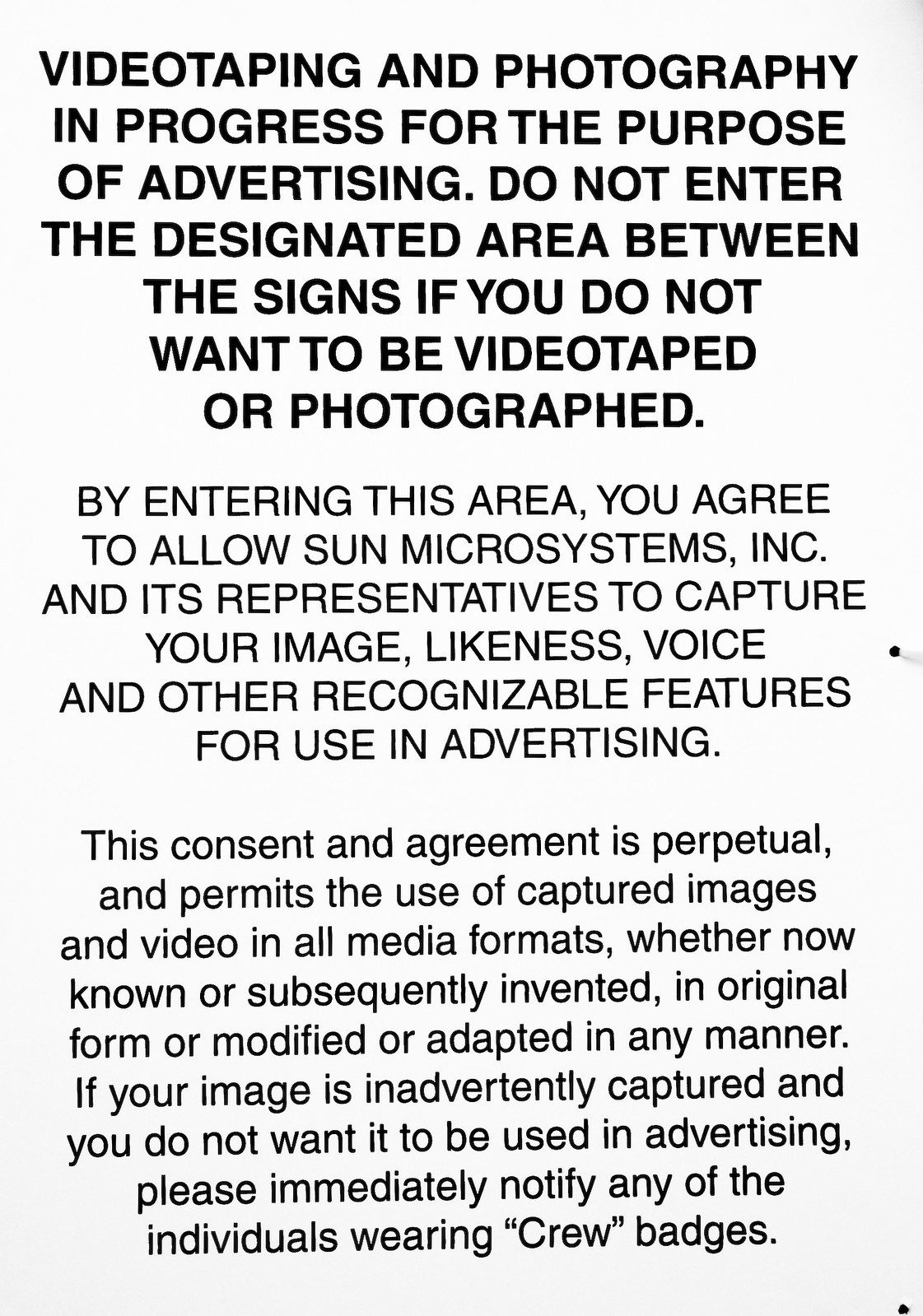This image depicts a close-up of a sign with a white background featuring three paragraphs of typed black text. The first paragraph, prominently bold and in all capital letters, states: "VIDEOTAPING AND PHOTOGRAPHY IN PROGRESS FOR THE PURPOSE OF ADVERTISING. DO NOT ENTER THE DESIGNATED AREA BETWEEN THE SIGNS IF YOU DO NOT WANT TO BE VIDEOTAPED OR PHOTOGRAPHED." The second paragraph, in slightly smaller but still bold text, reads: "By entering this area, you agree to allow Sun Microsystems Inc. and its representatives to capture your image, likeness, voice, and other recognizable features for use in advertising." The final paragraph, in standard lowercase lettering, explains the perpetual nature of this consent, allowing the use of captured images and videos in all media formats, whether existing or invented in the future, whether in original form or modified. It also advises those who do not wish their images to be used to notify any individual wearing a crew badge.